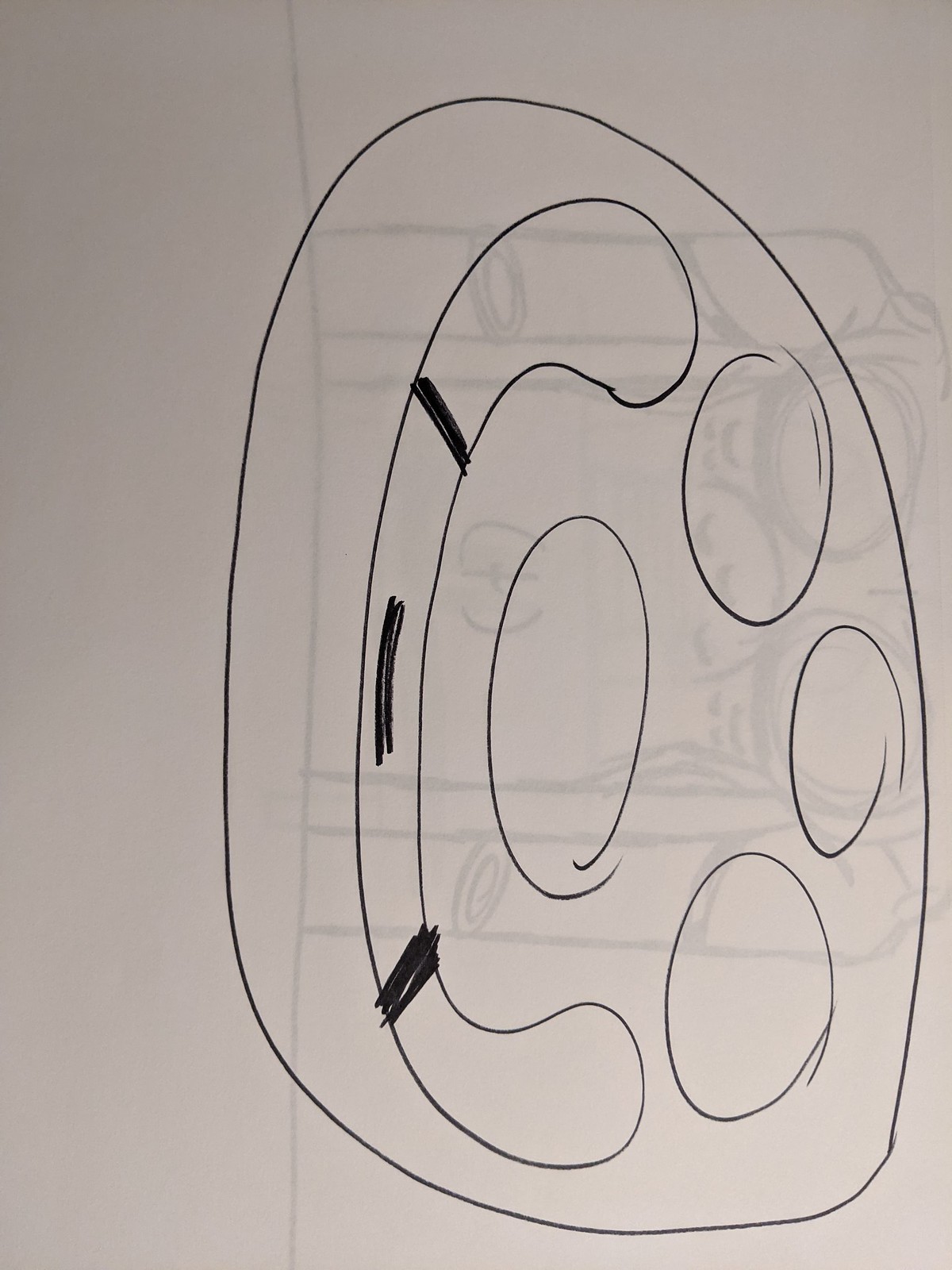The image showcases a rough sketch on a piece of paper oriented in portrait mode. The drawing, executed with either a pen or fine black marker, features an irregularly shaped oval dominating the center. On the right-hand side of the oval, there are four circles that appear to have been drawn hastily, with some of the circles not fully connected. These circles are grouped together in a 2x2 arrangement. Next to the circles, there is a curled shape that resembles a phone receiver, marked with two dark black scribbled stripes at each end and a single vertical stripe in the middle. Below this shape, faint gray lines are visible, possibly indicating marks from the other side of the paper bleeding through. Overall, the sketch conveys a sense of urgency and lacks intricate details.